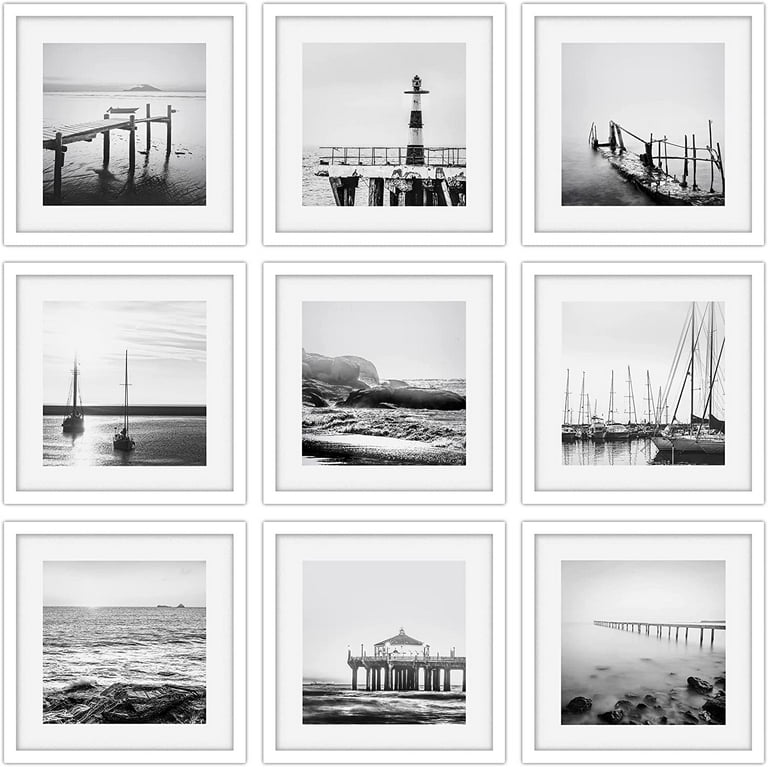This is a detailed black-and-white collage consisting of nine evenly-sized square photographs, each bordered by a white frame, arranged in a three-by-three grid resembling a tic-tac-toe board. The collection captures various beach and ocean scenes, including a mix of docks and piers—one featuring a structure possibly used for storage, another appearing collapsed into the sea, and others extending into the rolling waves. Notably, there's a striped lighthouse enclosed by a fence, and images showcasing both the serene and tumultuous aspects of the sea: from crashing waves along a rocky coastline to tranquil waters with boats sailing, some seen from a marina. The diversity and uniformity of these coastal scenes are elegantly unified by their consistent style and framing.